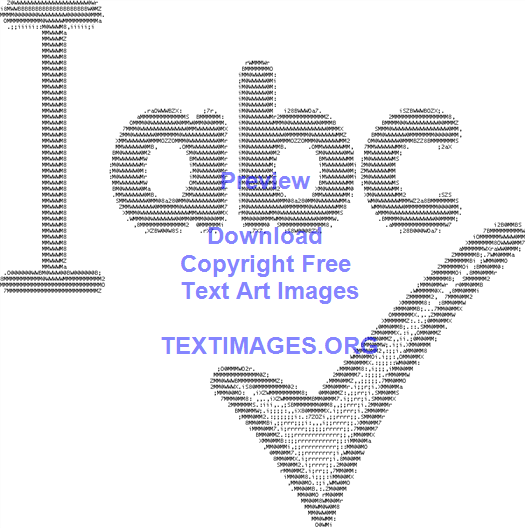The image is a computer graphic design featuring a completely white background. Prominently displayed on the left side is a large capital 'I' with rounded edges, followed by lowercase 'abc'. To the bottom right of 'abc' is a large checkmark. All these elements are composed of tiny black letters, numbers, and characters intricately arranged to form the larger shapes, giving the checkmark and the text darker and lighter shades. Overlaying the black and white text art is a watermark in blue that reads "Preview, Download, Copyright Free, Text Art Images, textimages.org."